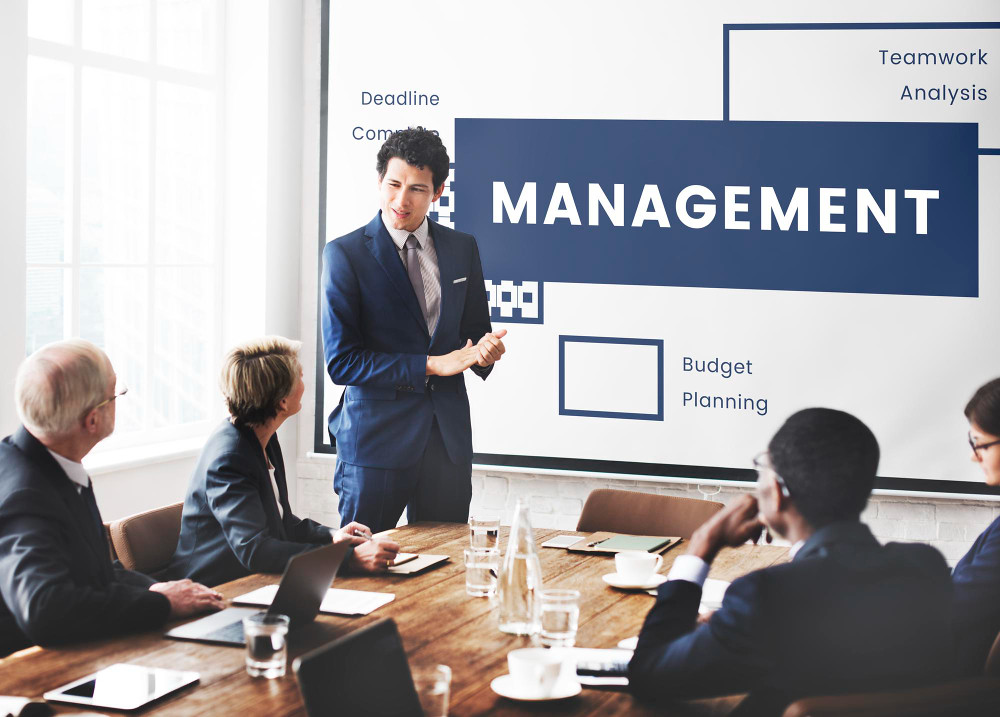The image captures a detailed scene inside a well-lit office meeting room, characterized by tall white-paned windows on the left, allowing natural light to pour in. Dominating the foreground is a large wooden conference table surrounded by brown chairs. Seated around the table are four individuals, with more suggested beyond the image’s edge due to visible tablets and other items. At the table's center lies a pitcher of water, complemented by glasses of water distributed among the participants. 

All attention focuses on a gentleman of Caucasian European descent standing at the front, dressed meticulously in a purple shirt and tie paired with dark blue pants and a matching suit jacket. He's positioned in front of a prominent whiteboard displaying a PowerPoint slide. The slide features a central blue rectangular banner with "MANAGEMENT" boldly inscribed in white. Above this, "Teamwork Analysis" is outlined in a blue-bordered white box, while below it, phrases like "Budget Planning" and "Deadline" are also visible.

To the left of the standing presenter sits a woman, also of Caucasian European descent, attired in a dark blue business suit, gazing attentively at the man. Beside her is an older, glasses-wearing gentleman with gray hair, also focused on the speaker. To the right sits another woman with brown hair and glasses, looking down at a document. Next to her, there's the rear view of an African-descendent man, dress-coded alike in a dark blue suit, thoughtfully resting his head on his hand as he listens.

The table is strewn with several laptops, clear glasses, and a white coffee cup with a saucer, indicating an active and engaged meeting setup.